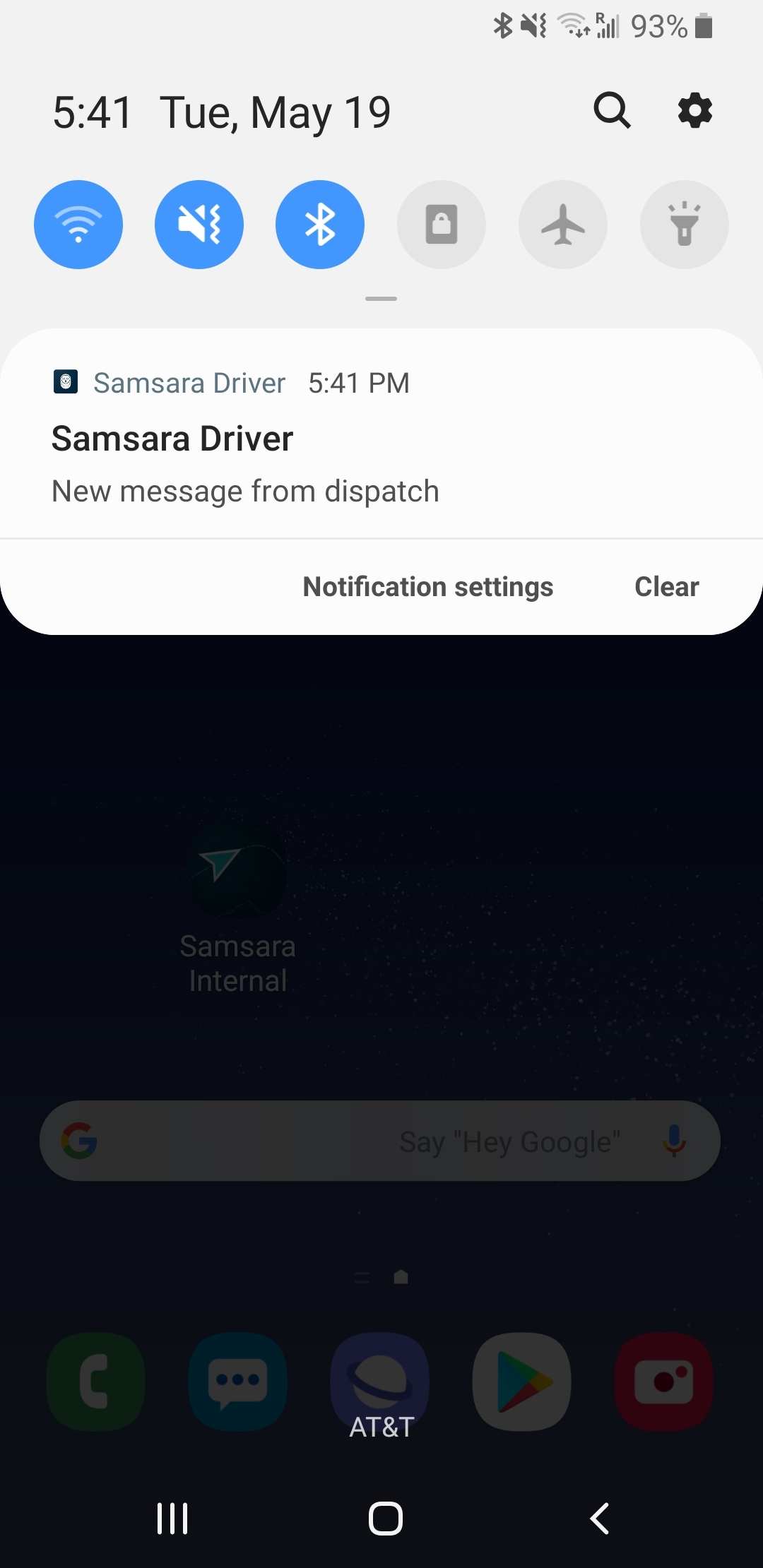In this image, we observe a smartphone screenshot with a variety of status indicators and interface features. In the top right corner, there are icons representing different functionalities: a beauty mode icon, a vibrate mode icon, a Wi-Fi signal icon showing one out of four bars, a network signal bar with four out of five bars, and a battery level indicator at 93%. The time on the device is 5:41, and the date is Tuesday, May 19th. Adjacent to these indicators are the search button and the settings button.

In the drop-down notification panel, we see several quick access icons, including Wi-Fi, sound, Bluetooth, phone lock, airplane mode, and flashlight. Among the notifications displayed are updates from the Samsung driver and a new message from dispatch. There are also options for notification settings and a "clear" button to dismiss the notifications.

At the bottom of the screen, a row of frequently used apps is visible, including the phone dialer app, messaging app, browser app, and the Google Play Store.